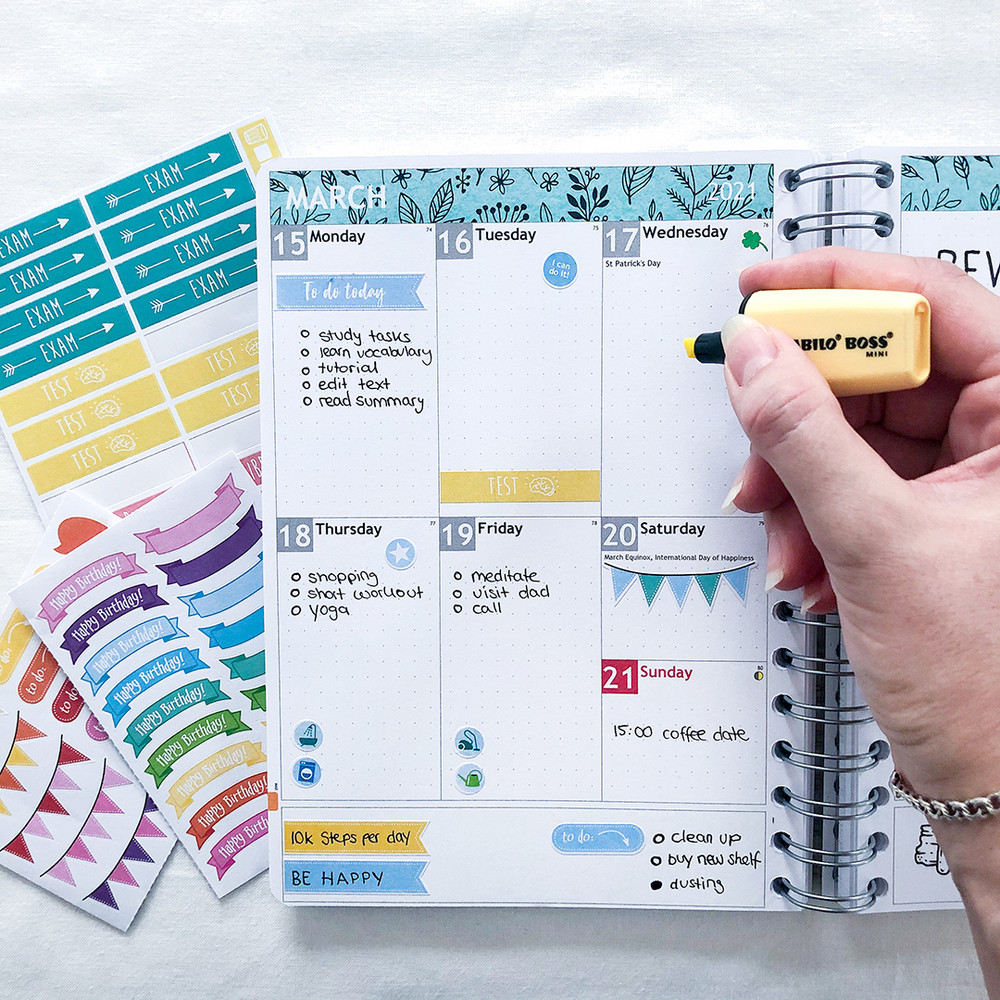The photograph captures a detailed view of an open day planner, specifically showcasing the month of March. The planner is structured with a week-per-page layout, organized into a 3x2 grid. Each section is meticulously arranged into days, with visible entries for March 15th and 17th, among other dates. Written tasks for March 15th include "study," "test," "learn vocabulary," "tutorial," "edit text," and "read summary." The planner features additional sections such as banners and a to-do list positioned at the bottom right, which includes tasks like "clean up," "buy a new shelf," and "dusting." A Caucasian hand holding a yellow highlighter hovers above the page, poised to mark or write on Wednesday the 17th. The image also subtly captures additional stationery items in the background, suggesting a committed and organized planning routine.